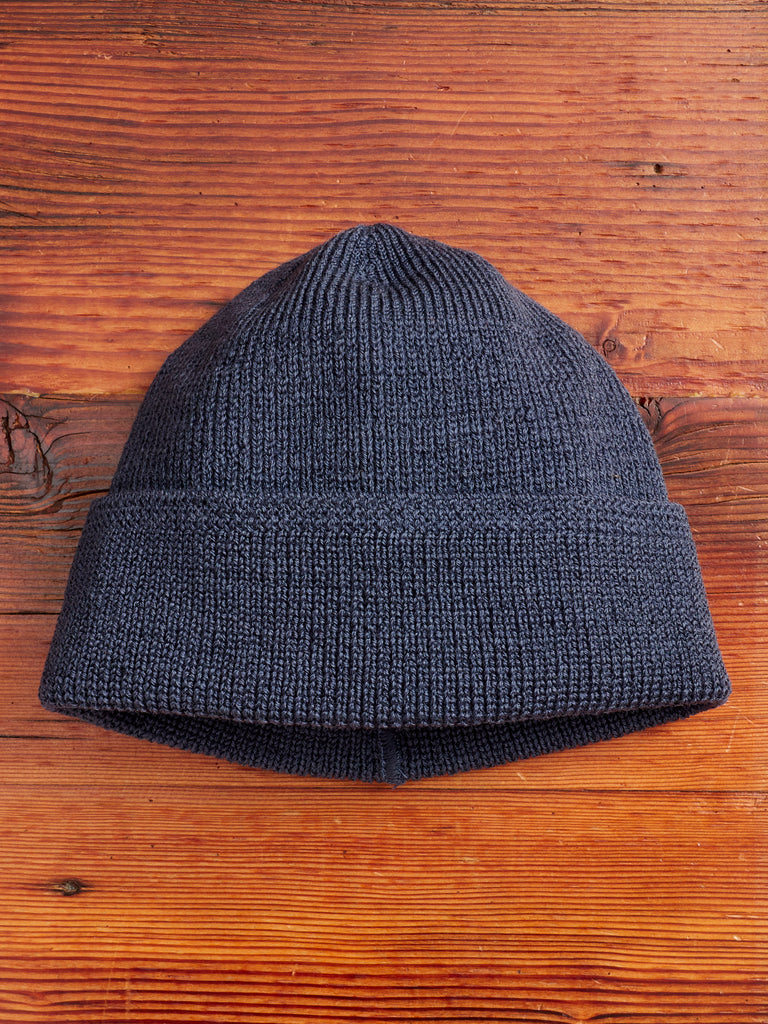The image features a simple, knitted winter cap placed on a wooden table. The cap, which is a shade of blue with hints of gray, has a traditional ribbed design and a folded-up bottom edge, typical of ski caps worn by fishermen or skiers. Its knitted texture is clearly visible, and it's laid flat in a relaxed position at the center of the frame. The background consists of a dark, orangey-brown pine table with prominent wood grain patterns running horizontally. A notable feature of the table is a brownish-black knot near the left-hand side, almost disappearing out of the frame. The image is minimalistic, focusing solely on the blue winter cap and the distinctive wooden surface.